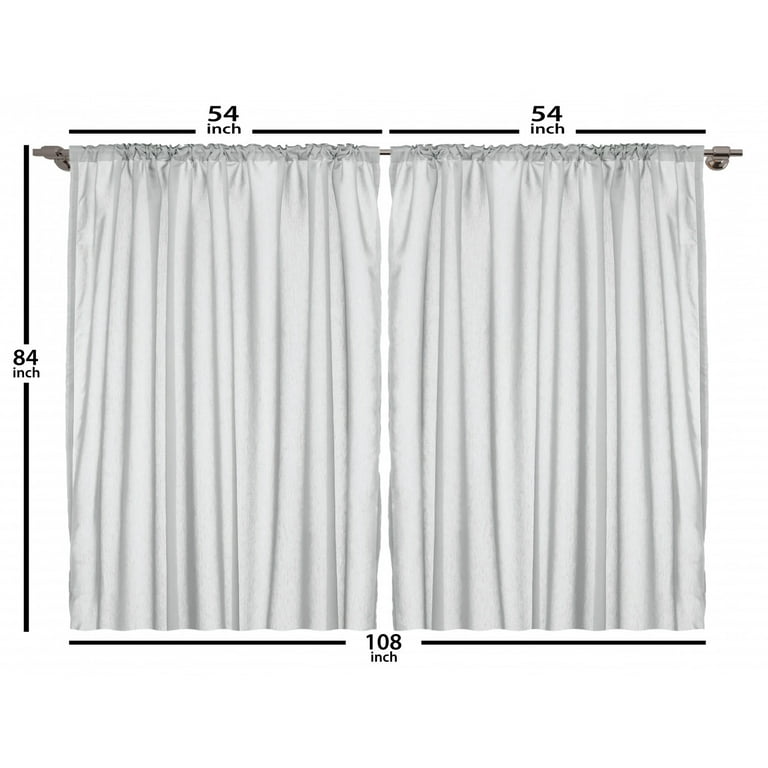This clear photograph showcases a pair of light gray curtains hanging on a copper-colored curtain rod against a white background. The curtains, meeting in the middle with a slight gap, are meticulously labeled with detailed measurements. Each curtain measures 54 inches wide and 84 inches high, making the combined width 108 inches. Black bars denote these dimensions: '54 inch' at the top indicates the width of each curtain, while '84 inch' on the left side illustrates their height. The bottom measurement, '108 inch', confirms the total width when both curtains are considered together. This image, likely intended for a retail website, emphasizes the precise dimensions and presentation of the curtains for potential buyers.